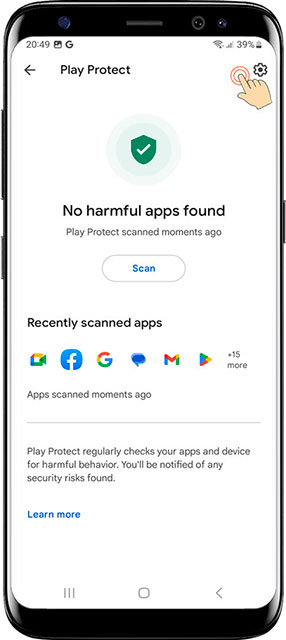In this image, we see a Samsung Galaxy S8+ mobile device displaying a Google Play Protect page. The time on the top left corner of the device screen is 8:49. Icons on the status bar include the Google icon, Wi-Fi signal strength indicator, and network signal strength indicator. The battery percentage is shown at 39%. 

The Play Protect page reports that the device has been scanned and no harmful apps were found. The recently scanned apps listed are Google Drive, Facebook, Google Messages, Gmail, the Play Store, along with 15 additional apps. Play Protect regularly scans apps and the device for harmful behavior and will notify the user of any security risks detected. Settings options are also visible on this page.